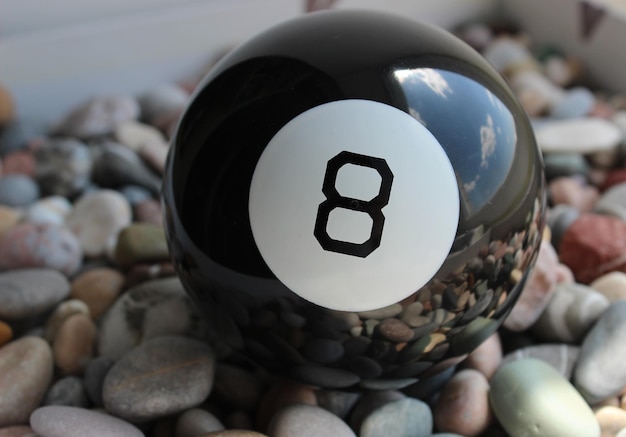In this detailed close-up color photograph, the focus is on a black 8 ball commonly used in pool games. The ball features a white circle in its center, within which the number 8 is prominently displayed. The glossy surface of the 8 ball vividly reflects its surroundings, including a sunny blue sky with white fluffy clouds and the multicolored stones on which it rests. The stones, which form a part of what appears to be outdoor landscaping, come in various colors—gray, red, white, pink, blue, and brown—and are of different shapes and sizes, primarily oblong and round. Although the background is blurry and slightly out of focus, a white wall or box structure is discernible, suggesting the stones and 8 ball might be contained within a specific area. The photograph captures the intricate details and reflective quality of the 8 ball amidst its vibrant, detailed environment.